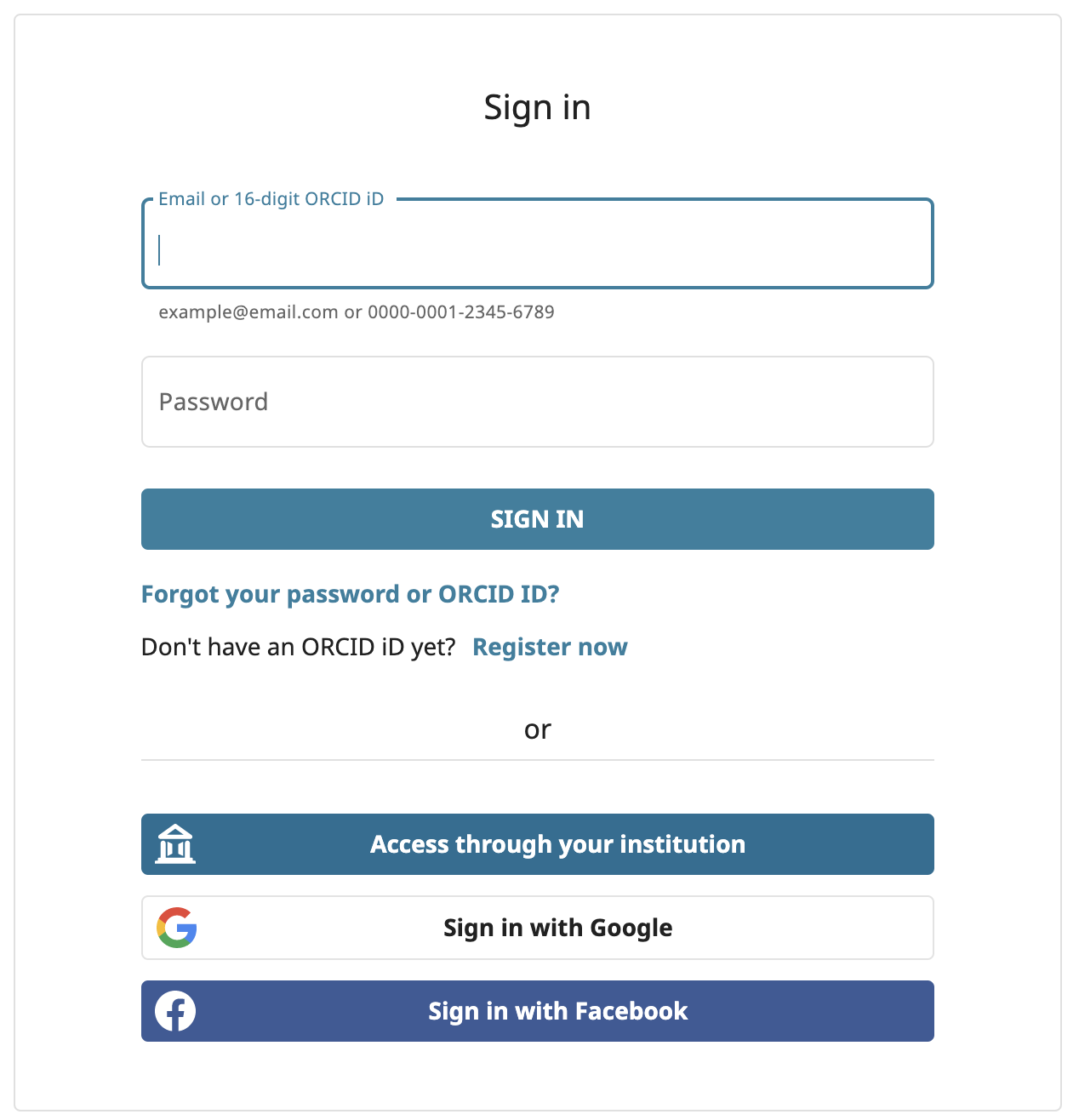A cropped screenshot of the ORCID sign-in page on either a mobile or tablet device is displayed. The interface is minimalist, featuring a white background and straightforward layout. At the top, it reads "Sign In," offering two input fields: one for either your email address or your unique 16-digit ORCID iD. Below this input field, examples are provided—‘example at email.com’ for the email and ‘0000-0001-2345-6789’ for the ORCID iD.

The subsequent field is for entering your password. Beneath the password box is a teal "Sign In" button, matching ORCID’s signature color. Directly below, links for "Forgot your password or ORCID iD?" and "Don't have an ORCID iD yet? Register now" are available for users needing additional assistance.

Further down the page, alternative sign-in options are presented, allowing users to sign in through their institution or via third-party services such as Google or Facebook. These buttons are color-coded and branded: a teal button for institutional access, a white button for Google with the Google logo, and a blue button for Facebook accompanied by the Facebook icon.